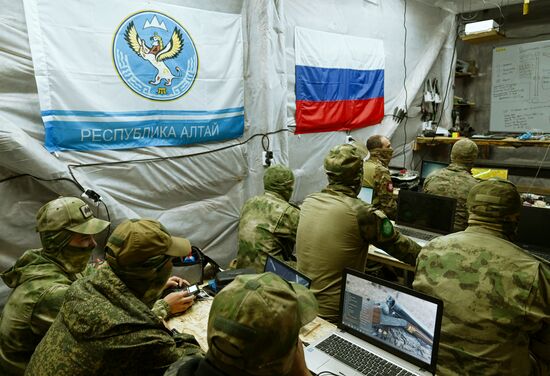The photograph depicts a secure intelligence tent of the Russian army, characterized by white tent walls. Prominently displayed on these walls are two flags: the Russian national flag, which is white, blue, and red, and another flag that features Cyrillic writing and a crest with a hawk or lion with wings and a crown. The room is filled with approximately eight soldiers, all clad in green camouflage uniforms, hats, and camouflage-patterned masks for concealment. They are seated in three rows at tables, each with a laptop, likely reviewing tactical data and terrain. A whiteboard with black writing and a white projector on a brown stand are also visible within the tent, suggesting an ongoing briefing or planning session. Black cables are seen trailing through the middle of the space, adding to the busy, high-tech atmosphere of the scene.